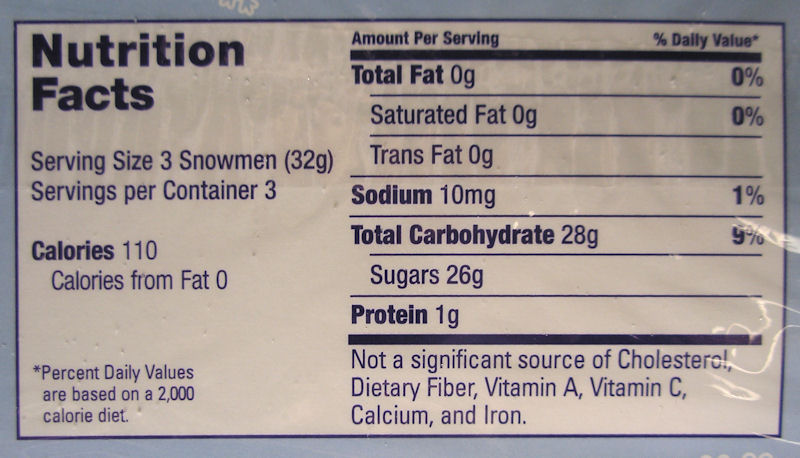In this photograph, we see a detailed nutrition label likely associated with a seasonal chocolate product themed around snowmen, suggesting it is marketed for the Christmas season. The label specifies that the serving size is three snowmen, with a total of three servings per container. Each serving contains 110 calories. Nutritional details are meticulously listed: total fat, saturated fat, trans fat, sodium, and other relevant dietary metrics, with the reminder that the percentage daily values are based on a 2,000-calorie diet, written in dark blue. Noteworthy is the disclaimer that the product is not a significant source of cholesterol, dietary fiber, vitamin A, vitamin C, calcium, and iron. The label is bordered in light blue, with a white background enhancing readability.